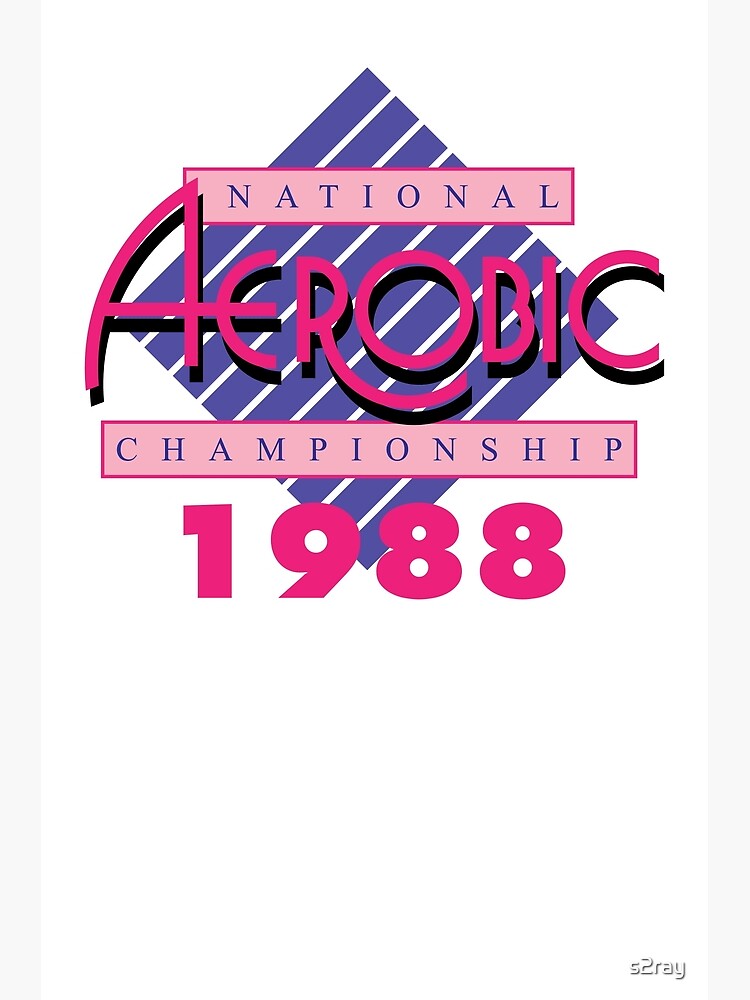The image appears to be a digitally produced logo on a primarily white background, with touches of off-white along the edges. Prominently featured in the center are purple bars arranged to form a square-like structure made up of nine bars. At the top of the logo, there is a bold pink box with a darker pink outline containing the word "National" in blue font. Below this, another pink box with a dark pink outline holds the word "Aerobic" in uppercase Art Deco red letters with a black shadow. Further down, a third pink box with a dark pink outline showcases "Championships" in blue letters. The year "1988" is displayed in thick, bold pink or magenta lettering directly beneath the boxes. In the lower right-hand corner of the logo, the name "S2 Ray" is printed in white. The overall color scheme emphasizes shades of pink, magenta, and purple, giving the logo a vibrant, retro feel reminiscent of a vintage advertisement or poster for the "National Aerobic Championship 1988."